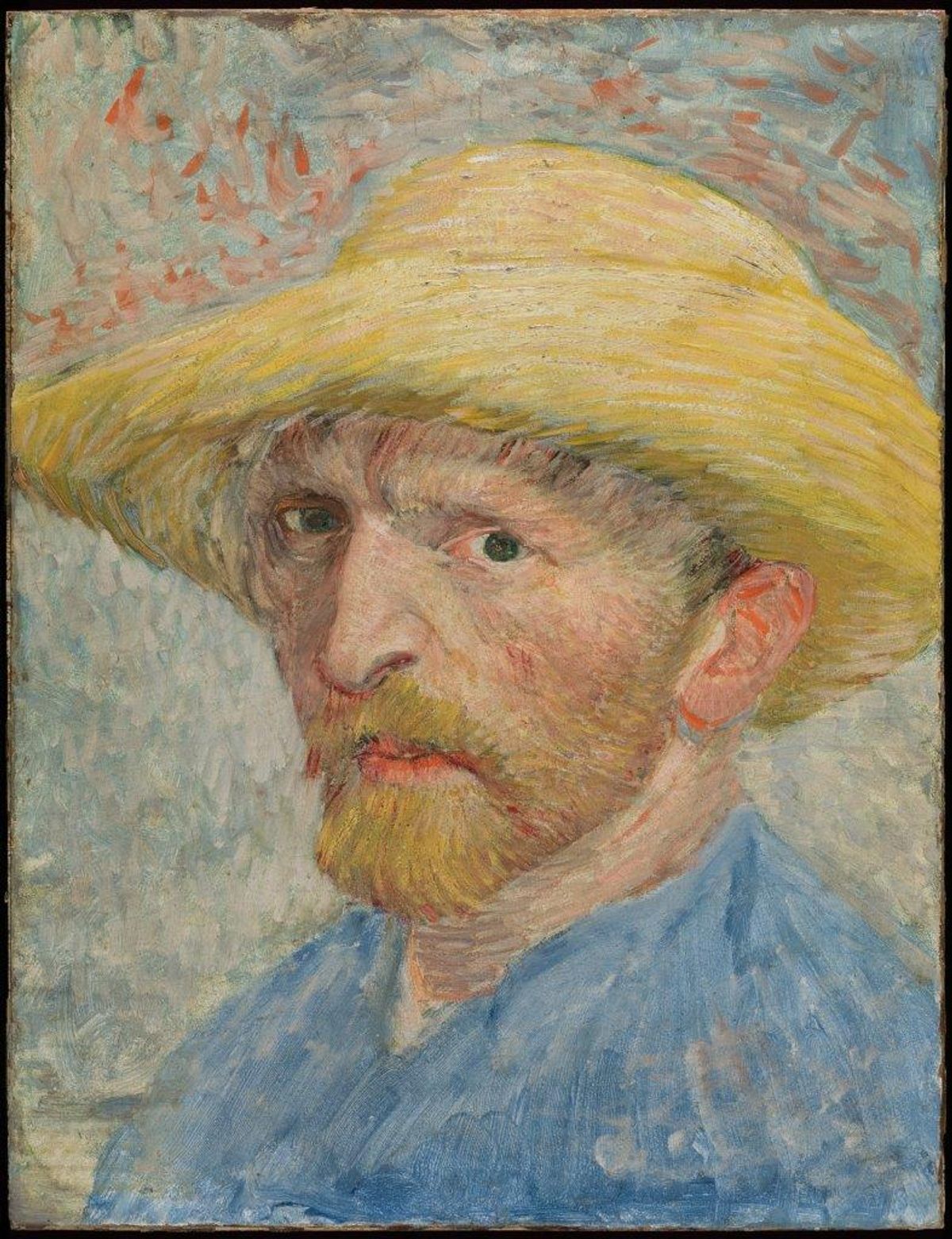This painting is one of Vincent van Gogh's self-portraits, showcasing his distinctive impressionist-inspired yet uniquely personal style. The artwork, executed in oil, features Van Gogh in a blue-collared shirt, possibly with a white undershirt peeking through. His face, pale with intricate separations of color rather than a smooth surface, is slightly tilted to the right, with his gaze directed inquisitively toward the viewer. Van Gogh is depicted with a blonde beard that is not overly thick but frames his face alongside a matching mustache. He is adorned with an eccentric straw hat that exhibits varying shades of yellow and light accents, and its brim intriguingly curves away from his head. His hair, visible in front of his left ear and alongside his playful straw hat, has a reddish hue. Van Gogh's green eyes, vivid against his complexion, add life to the portrait. The background is a mix of dark grays, greens, and intermittent whites, with reds enhancing the upper portion, adding depth and contrast to the composition. The painting is framed in black, against a white wall, highlighting Van Gogh's contemplative and introspective expression, characteristic of his renowned self-portraits.